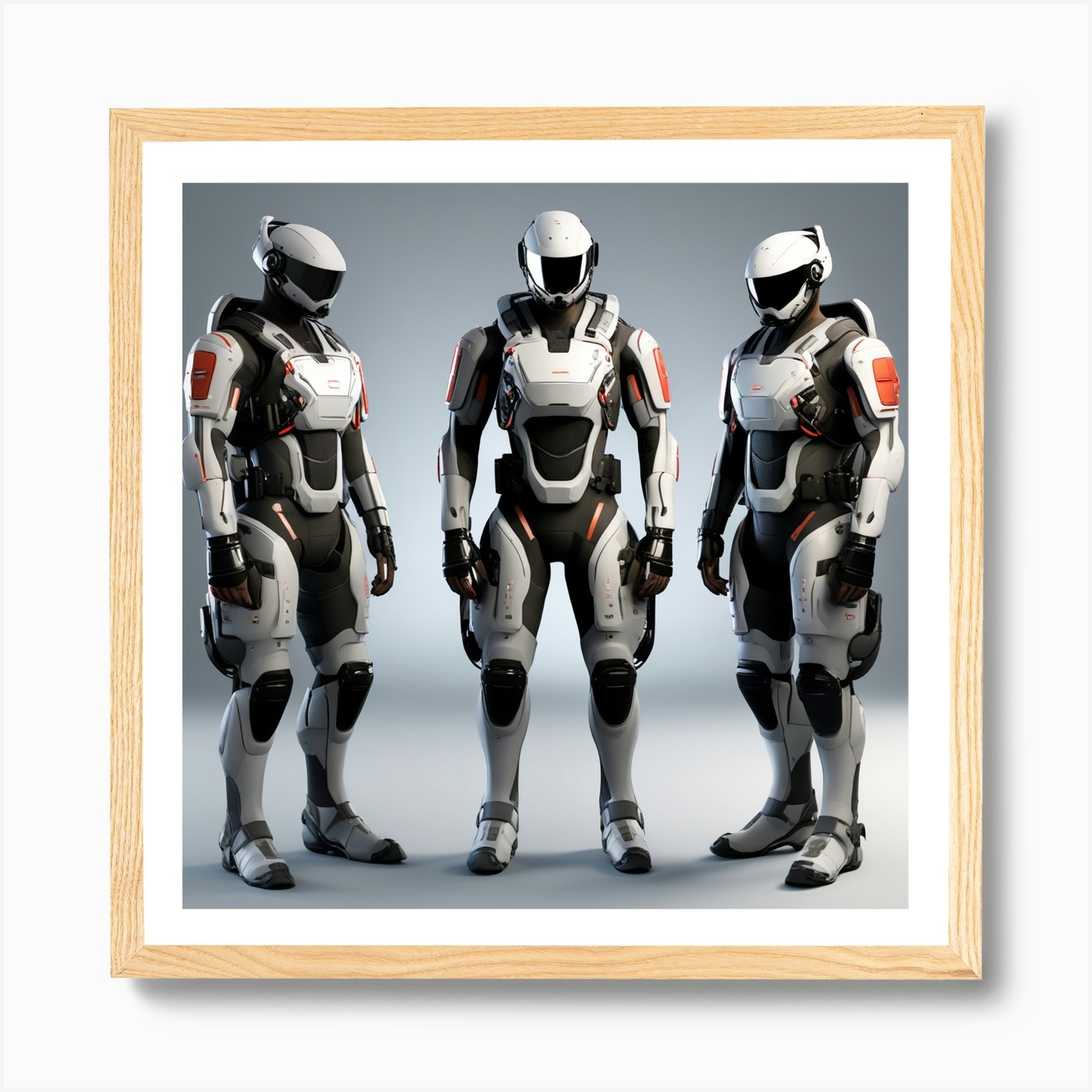This image, enclosed in a square, light wood-colored frame and adorned with a white border, features three figures clad in futuristic space suits. Resembling stormtroopers but distinct, these figures might be robots or humans in robotic-like armor. The suits cover them completely from head to toe with a blend of white and black protective gear, possibly made of plastic or polymer. Each figure's helmet, reminiscent of a motorcycle helmet, includes a black visor shielding their eyes. The background of the picture graduates from a dark to a lighter gray as it moves downward. The three figures are oriented differently: the one on the left faces right with a slight tilt, the middle one looks straight ahead, and the figure on the right faces left, also with a slight turn. Their gear features details such as black gloves, black knee caps, and gray side and leg pieces, with distinct items like silverish boots and a noticeable red area on the right shoulder of the leftmost figure.